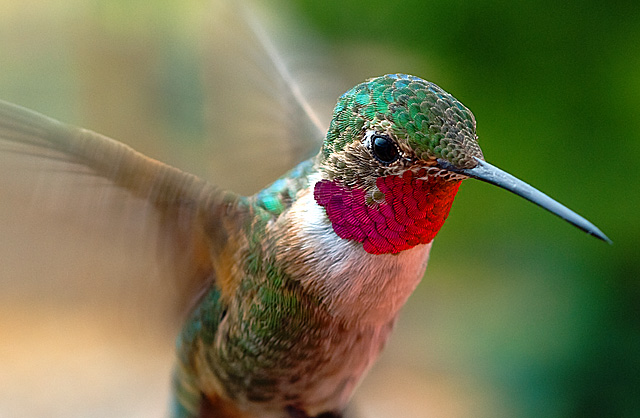This horizontal, close-up photograph captures a stunning, vibrant hummingbird in midair against a blurred background of green, brown, and hints of gold. The focal point of the image is the hummingbird's intricately detailed head, which showcases a captivating palette of colors: a vivid green crown, a striking red throat, and intermixed patches of brown and white below. The bird's sharp, elongated beak appears almost blue, and its black eye is distinctly visible, exuding a sense of life and motion. While the wings are mere blurs due to their rapid movement, suggesting the bird is in flight, the body remains crisp, highlighting the intricate feathers transitioning from the red throat to the brown-green belly. The blurred background further emphasizes the bird's dynamic presence, giving it an ethereal, almost surreal quality. This exquisite ruby-throated hummingbird is beautifully frozen in a moment that showcases its grace and the amazing speed of its wings.